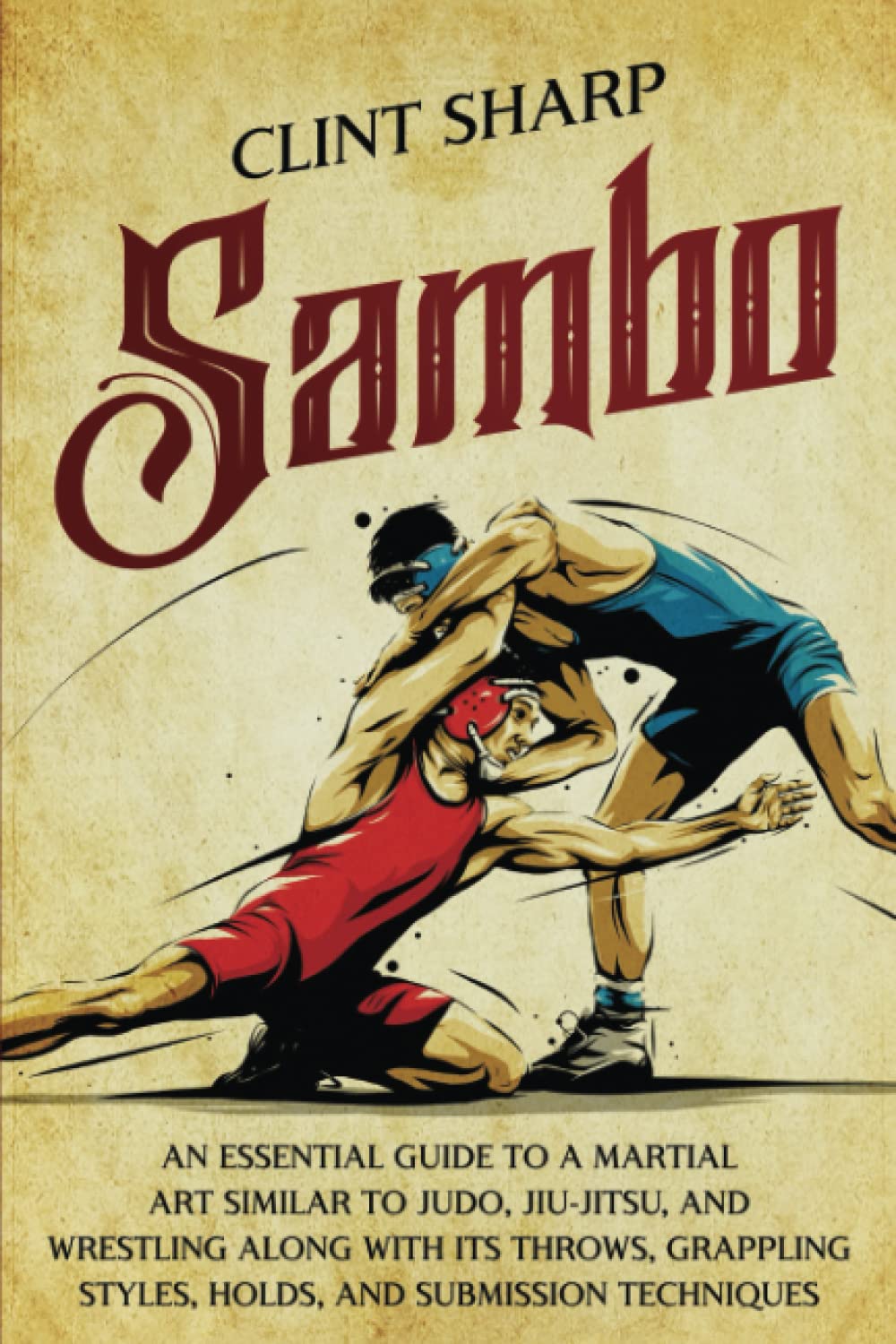The image depicts a book cover with a light beige background that resembles weathered parchment, featuring an illustration of two wrestlers in action. The wrestler on the left wears red jersey shorts and headgear, while the one on the right is dressed in blue jersey shorts and headgear. The top of the cover showcases the title in black text, "Clint Sharp," angled slightly upward toward the right, followed by the word "Sambo" in bold red letters. Below the illustration, black text states, "An essential guide to a martial art similar to Judo, Jiu-Jitsu, and wrestling, along with its throws, grappling styles, holds, and submission techniques."